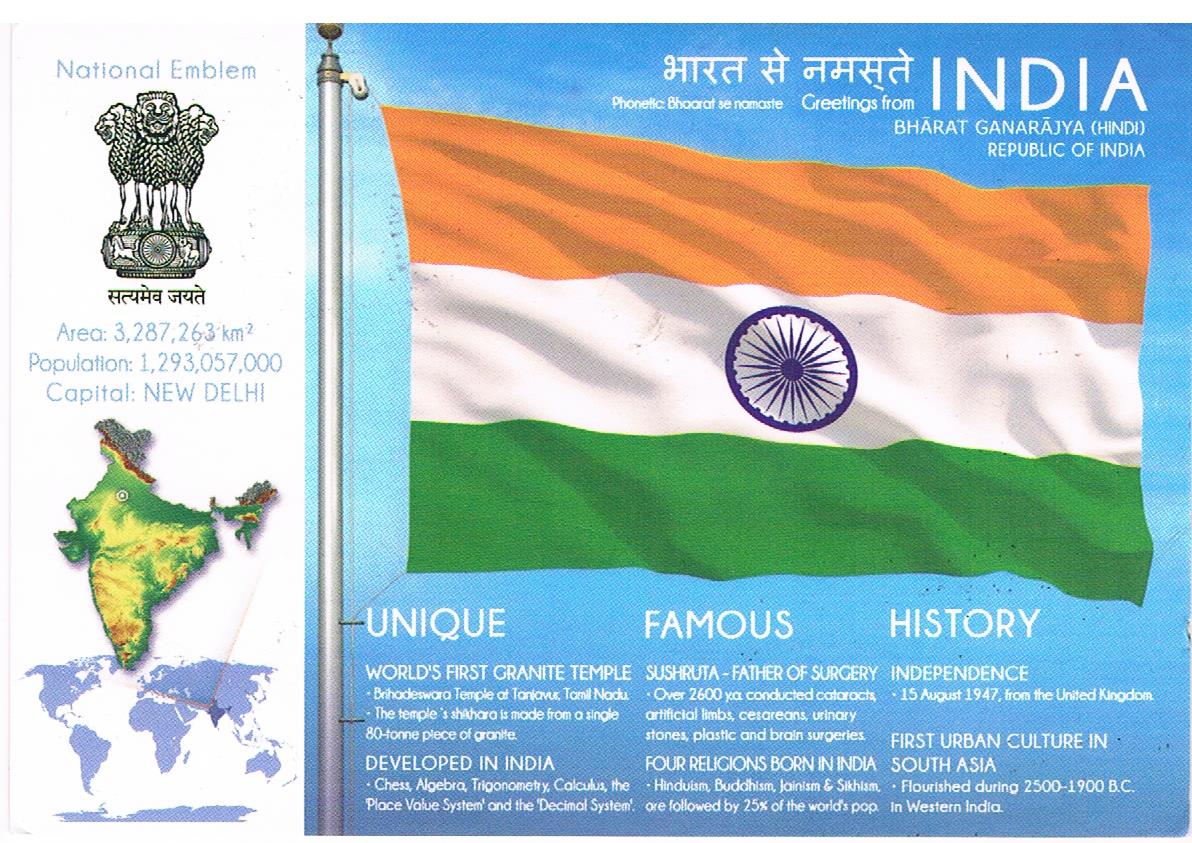The image is a detailed, landscape-oriented graphical representation of India, featuring both its national flag and an assortment of notable information about the country. The leftmost fourth of the image consists of a vertical white banner displaying India’s National Emblem — a stone statue with three lions facing different directions, and text in blueprint style that reads "Area: 3,287,263 km²", "Population: 1,293,057,000", and "Capital: New Delhi". Below this, a map shows India in relief with geographical elevation indicated through color gradients ranging from green to brown, and another map depicts India’s location on the globe.

To the right, set against a blue background, is a silver flagpole with the Indian flag waving, which has three horizontal stripes: saffron (top), white (middle), and green (bottom). At the center of the white stripe is a blue Ashoka Chakra, a 24-spoke wheel. Above the flag, white text reads "India, Bharat Gana Rajya (Hindi), Republic of India".

Below the flag, various achievements and facts are listed in white text. “Unique” mentions the world’s first granite temple. Further details under “Developed in India” include innovations such as chess, algebra, trigonometry, calculus, the place value system, and the decimal system. Under “Famous,” it highlights Sushruta, known as the father of surgery, who over 2,600 years ago, conducted various surgical procedures including cataract, cesareans, and brain surgeries. Four religions — Hinduism, Buddhism, Jainism, and Sikhism — born in India, are noted as being followed by 25% of the world's population. Historical information states India’s independence from the United Kingdom on August 15, 1947, and highlights the first urban culture in South Asia which flourished in Western India from 2500 to 1900 BC.

The detailed composition emphasizes the blend of India’s historical significance, contributions to various fields, and geographical data, offering a comprehensive snapshot of the nation.